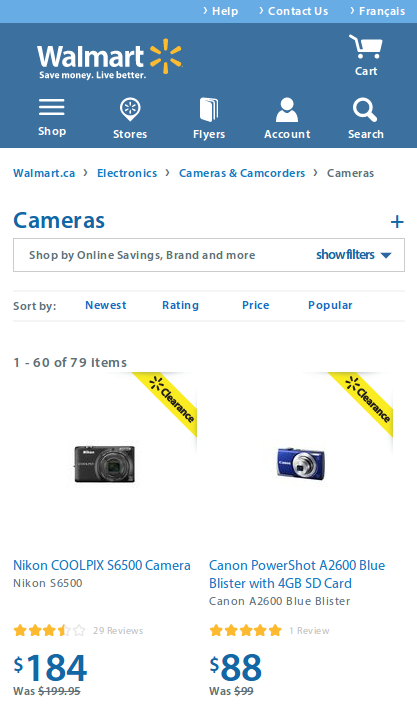The screenshot displays a segment of Walmart's website, starting with a thin light blue header at the top. The top-right corner houses a menu containing options for Help, Contact Us, and Language Selection, which currently displays French. Below this thin panel is a broader, darker blue banner featuring the Walmart logo and name on the left side. Underneath this banner, several icons are lined up, including options for Shop, Stores, Flyers, Account, and a Cart icon just above the Search bar.

Further down, the webpage showcases a collection of selectable categories such as walmart.ca, Electronics, Cameras & Camcorders. The current display indicates that the user has navigated to the Camera section. Below the Cameras category, there is a search function available to help users find specific brands or online deals, with options to sort the results by Newest, Price, or Popular.

The main content area presents two highlighted camera brands. The first product is a Nikon Coolpix camera, prominently priced at $184 in a large font, with the original price of $199.95 shown below in a smaller, struck-through font. The second product is a Canon Powershot camera, currently priced at $88, down from its original price of $99, with the discount clearly indicated in a similar manner.